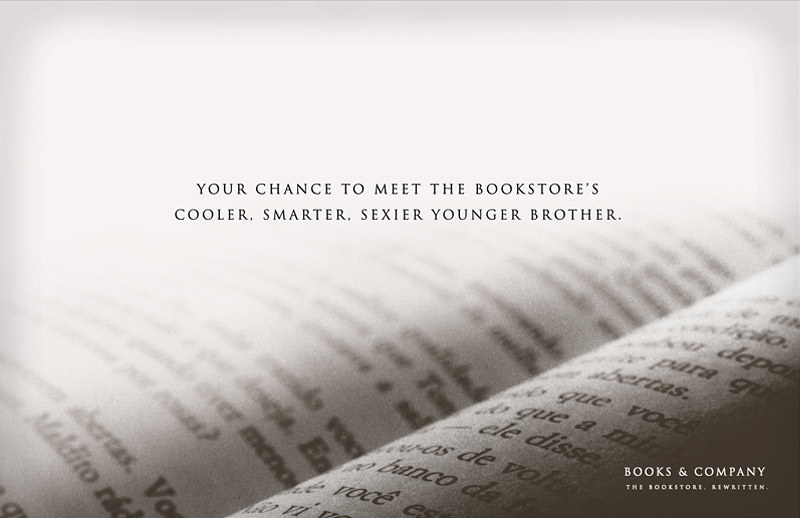The advertisement is a black and white image showcasing a close-up photograph of an open book, focusing on the center where the pages meet. The detailed texture of the book's text is visible but unreadable, creating a visually striking background. The image fades from the detailed book in the middle towards a lighter white gradient, particularly prominent in the top part, adding a dramatic, almost ethereal effect. Overlaying this are bold black letters across the center that read: "Your chance to meet the bookstore's cooler, smarter, sexier, younger brother." This statement is the focal point of the ad, drawing immediate attention. In the bottom right corner, in smaller white text, the ad subtly presents the brand: "Books and Company, the bookstore rewritten." This ad, characterized by its grainy texture and sophisticated monochrome palette, creates a modern and intellectual appeal.